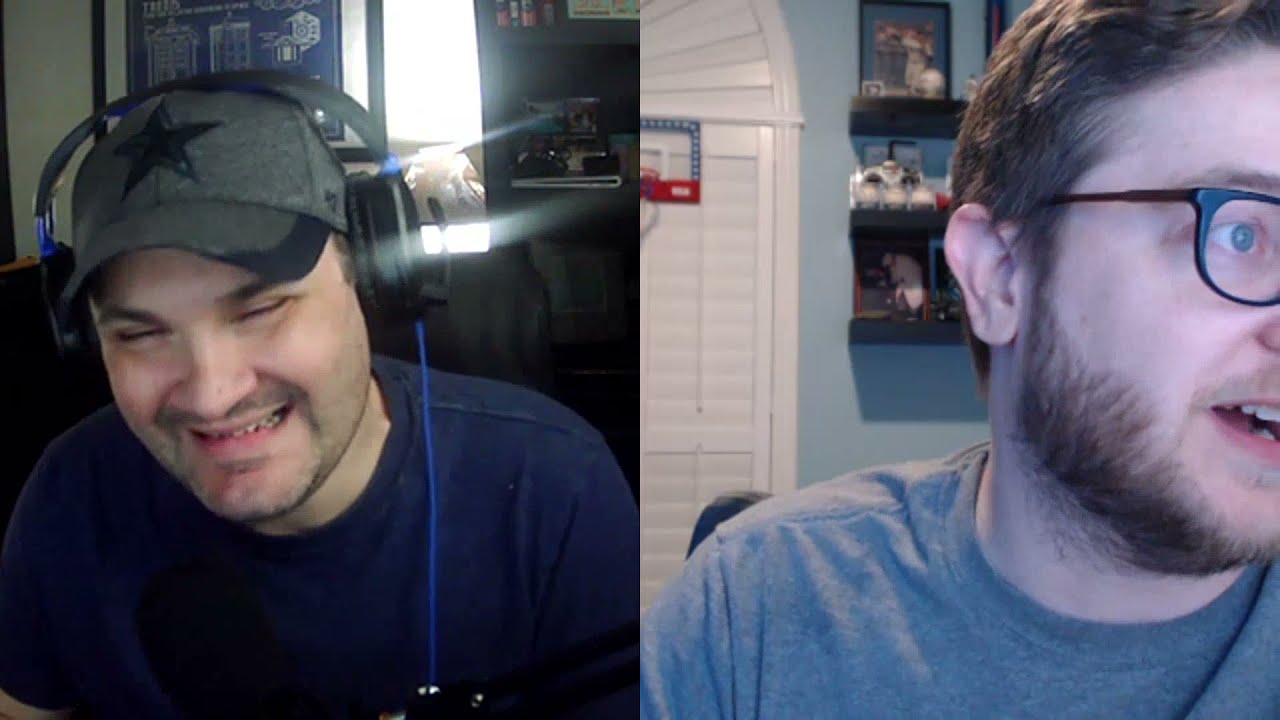The split image captures a video call between two young men, each in their respective bedroom environments. On the left, the man wears a dark gray baseball cap featuring a darker gray star, over-the-ear headphones with a visible cord extending from the left side, and a dark blue t-shirt. He is smiling broadly, with his mouth slightly open and eyes closed, as sunlight streams through a window behind him, giving his space a brighter ambiance. The man on the right appears close to the camera, sporting black-rimmed glasses, short brown hair, a short beard, and a grayish-blue crew-neck t-shirt. His gaze is directed away from the camera toward the right edge of the frame. Behind him, an arched white doorway stands next to a pale blue wall with shelving and a closet door featuring a basketball hoop.